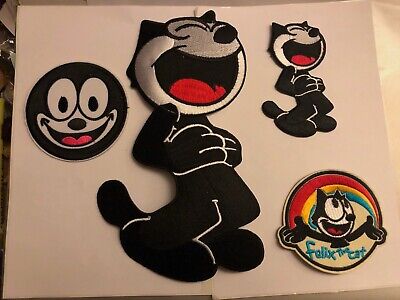This image showcases a collection of Felix the Cat patches on a white background, which could be used for items like jackets, purses, or book bags. The central focus is a large patch of Felix the Cat's full body, with his arms hugging his torso and mouth wide open in laughter, showing his red tongue. This same design is repeated on a smaller patch to the right. In the top left is a circular patch featuring just Felix's face, outlined in black with a white interior and a red tongue, giving a cheerful expression. The bottom right of the image displays another patch showing Felix from the chest up with his arms outstretched, accompanied by a rainbow arching from one hand to the other behind him. Below Felix, "Felix the Cat" is written in blue text.